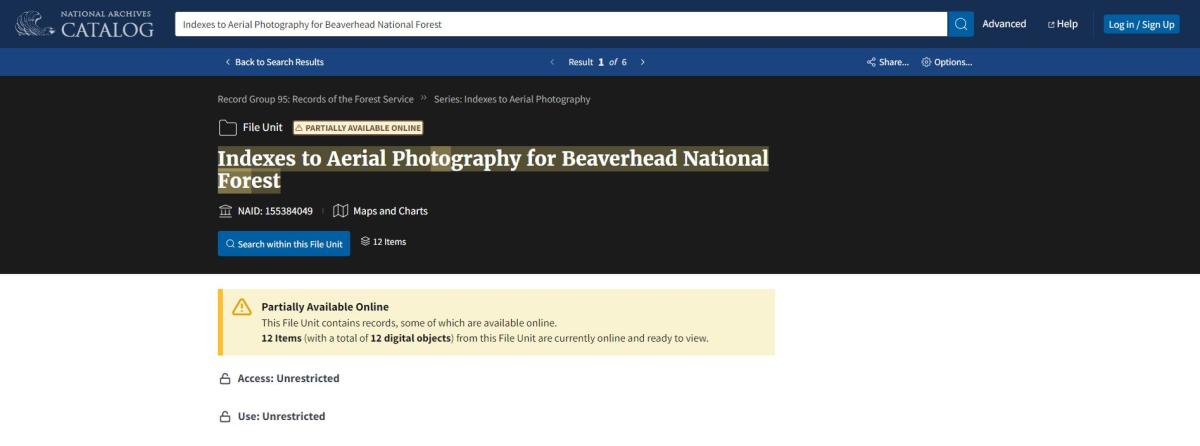The homepage of the National Archive Catalog is prominently displayed, featuring a sleek interface with a dark blue header. At the top, a pristine white search bar displays the query "Indexes to Aerial Photography for Beaverhead National Forest." Adjacent to the search bar is a blue magnifying glass icon for initiating the search, alongside additional buttons labeled "Advanced," "Help," and a distinctive "Login/Sign Up" button.

Beneath the header, a navigation option "Back to Search Results" is present, indicating the current display of "Result 1 of 6." The description below includes "Record Group 95, Records of the Forest Service," and further specifies the series as "Indexes to Aerial Photography." The status "Partially Available Online" is clearly highlighted, indicating the accessibility of some records online.

Highlighted in yellow, the title "Indexes to Aerial Photography for Beaverhead National Forest" stands out, alongside its National Archives Identifier (NAID) of 155-384-049. The section titled "Maps and Charts" includes a blue button for "Search Within this File Unit," which encompasses 12 items. Another yellow label reiterates "Partially Available Online," clarifying that some records are immediately accessible online—12 items with a total of 12 digital objects are fully available for viewing.

The information about access and usage rights is boldly emphasized with “Access Unrestricted, Use Unrestricted.” The overall webpage design is clean and user-friendly, with a white background dominating most of the page, complemented by a dark blue header and a section featuring a black background with white text, providing clear and easy navigation options for users.